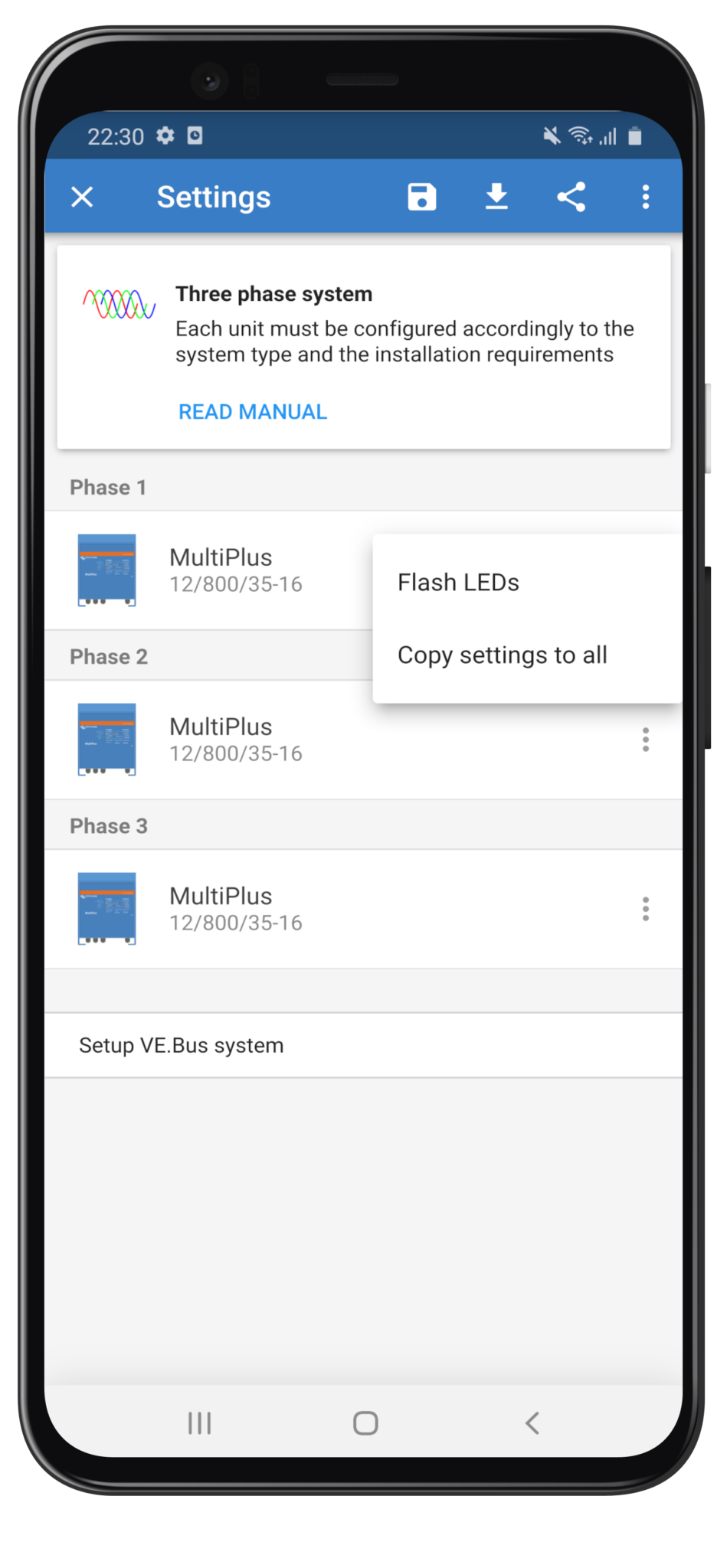The image depicts a smartphone screen, showcasing a detailed interface. At the top of the screen, the time is displayed as 22:30, accompanied by icons for settings (gear icon), notifications (square icon), a muted microphone (microphone with a line through it), Wi-Fi signal, service connection, and battery status.

Below that, a blue bar features a left-aligned white "X," the word "Settings," and various icons including a down arrow and a three-dots menu.

Continuing further, there is a white box containing the text: "Three-phase system. Each unit must be configured according to the system type and the installation requirements. Read manual," followed by a blue button.

The section below lists three phases:
1. Phase 1: MultiPlus 12-800 35-16, accompanied by a partially obscured blue image.
2. Phase 2: MultiPlus 12-800 35-16.
3. Phase 3: MultiPlus 12-800 35-16.

At the very bottom, the options "Setup VE Bus system" and "Flash LEDs" along with "Copy settings to all" appear to have interactive features, suggesting recent user interaction. The overall design consists of blue and gray bars with black text on a predominantly white background.